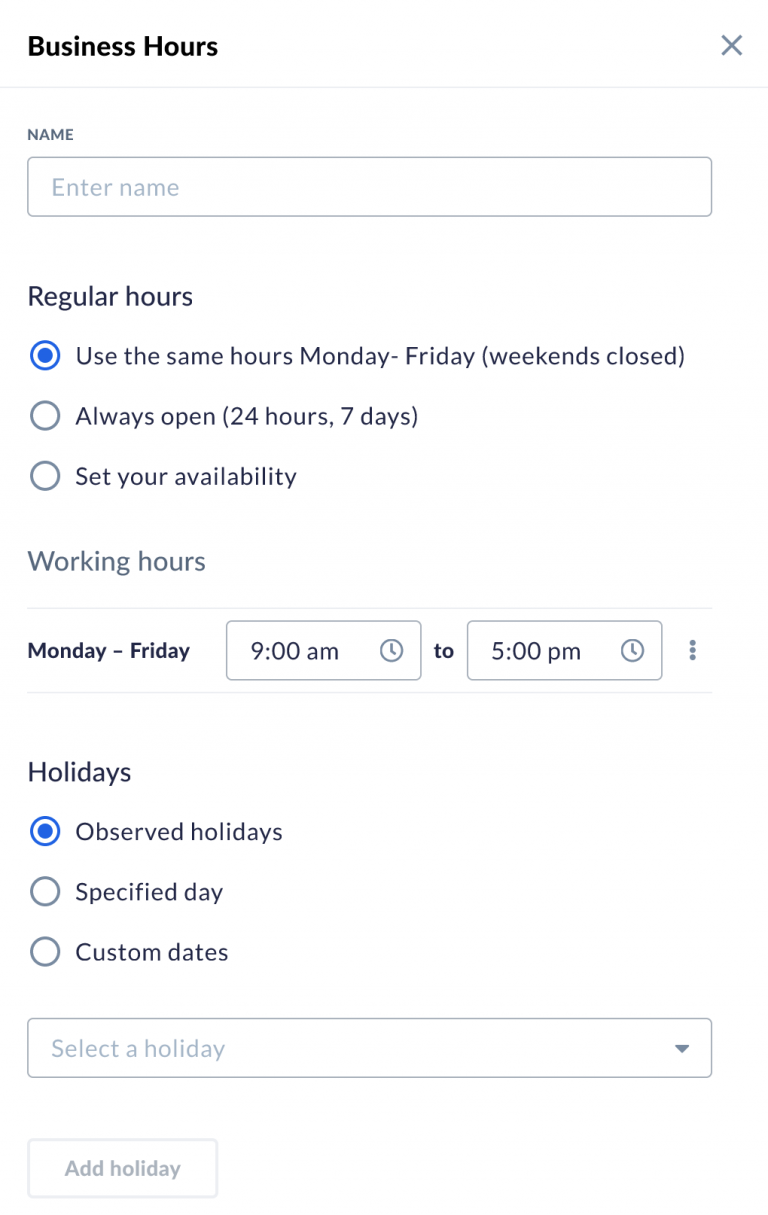The image displays an interface for setting business hours. It features a simple white background with text and interactive fields. On the top left, "Business Hours" is prominently displayed. On the top right, there is a small 'X' icon.

Below, there is a field labeled "Name" with placeholder text "Enter Name". Farther down, the section for hours distribution appears with three options, each accompanied by a radio button. The selected option, filled with blue, is labeled "Use the same hours Monday through Friday, weekends closed". The other two choices are "Always open, 24 hours 7 days" and "Set your availability".

Beneath these options, there is a "Working Hours" section specified for Monday through Friday, with time fields currently set from 9 a.m. to 5 p.m.

Further down, there is a "Holidays" section. The option "Observe holidays" is ticked, and the interface allows for additional specifications with "Specified days and custom dates." The dropdown menu labeled "Select a holiday" and an "Add Holiday" button with a white background and gray outline are available for user input.

Currently, the name field is empty, but the business hours are configured to 9 a.m. to 5 p.m. from Monday to Friday with holidays observed. The interface appears designed for setting and customizing business hours online.